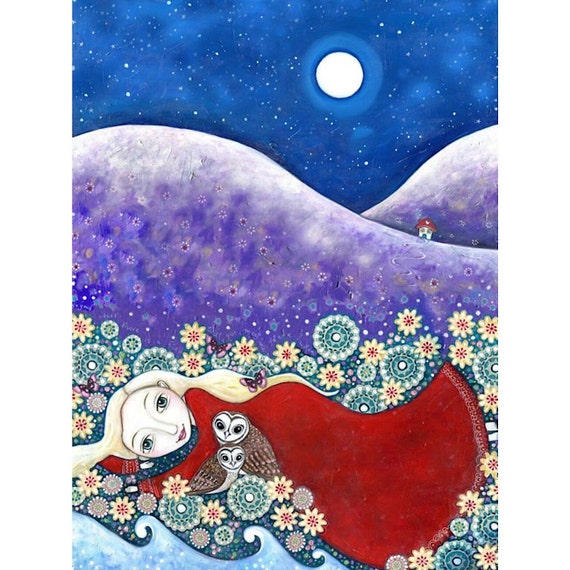In this vibrant, nighttime illustration reminiscent of a children's book, a large, bright full moon illuminates the dark blue sky, dotted with twinkling stars. The serene backdrop features two rolling, purple-colored mountains. At the base of the furthest mountain is a whimsical house with a mushroom-like shape, adorned with a brown roof, white exterior, and a blue door. 

Closer to the foreground, colorful flowers in shades of green, white, blue, pink, and red blanket the landscape. Nestled in this floral bed is a young lady, possibly a princess, lying on her side. She wraps herself in a long, red dress, her hair a striking white, with a butterfly perched on it. Her large, wide-set eyes gaze peacefully into the distance, framed by a round face, small nose, and thin lips. In front of her, two owls - a brown mother owl and a smaller baby owl - keep her company under the starlit sky.